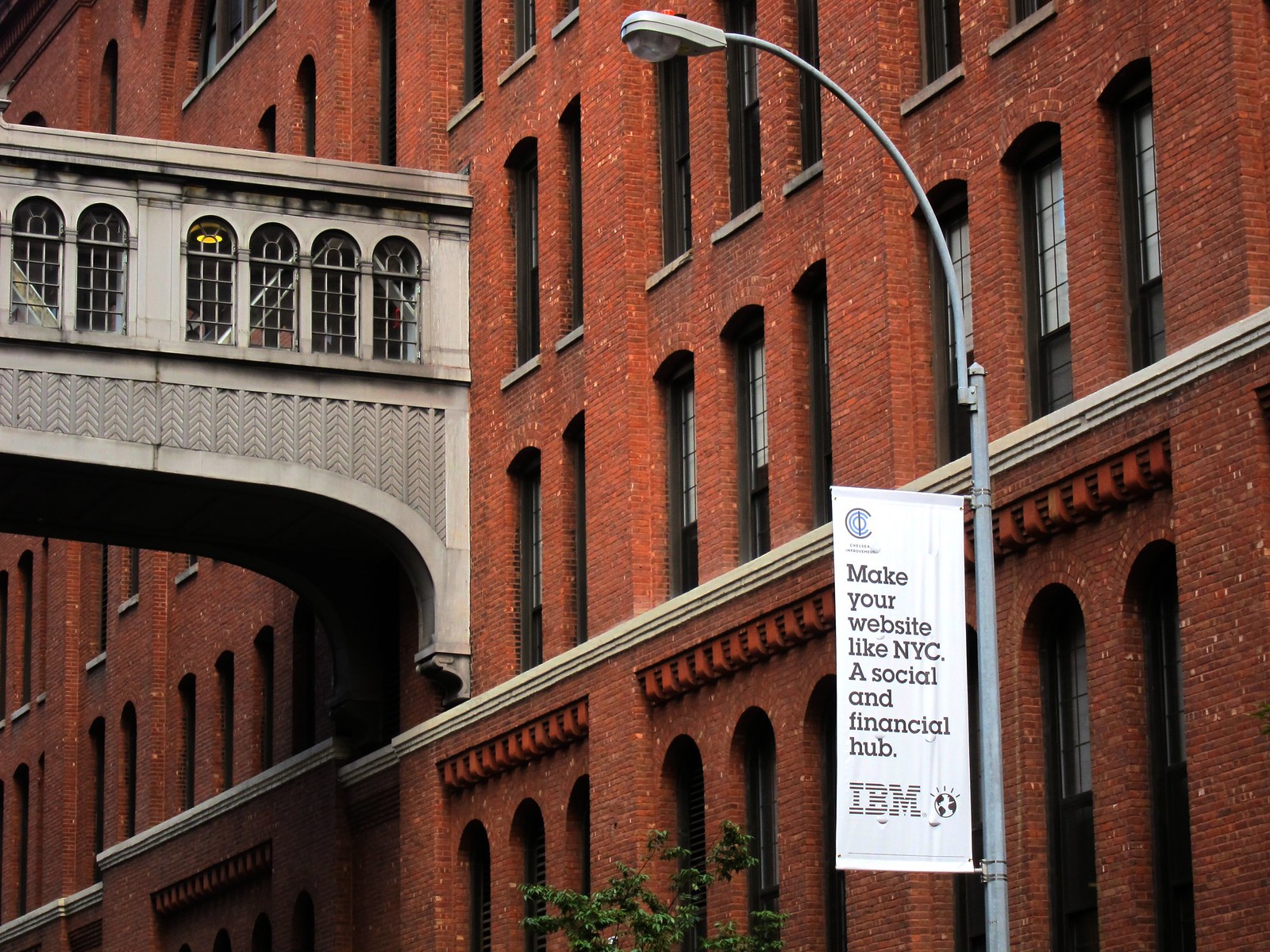This image captures an upward view of a large red brick building that appears to be around five stories tall, though only a portion is shown. The building features many arched windows with black bars, and behind these windows, you can see arch-shaped cutouts adding architectural detail. A gray pedestrian walkway, possibly connecting to another building, extends from the side. In the foreground, off to the right, there's a light pole curving over what seems to be a street or sidewalk. Attached to the pole is a white banner that reads in black lettering, "Make your website like NYC, a social and financial hub," followed by "IBM" at the bottom. The top of a small tree is also visible, providing a bit of natural contrast to the urban scene. The overall atmosphere suggests a newer, well-maintained city setting.